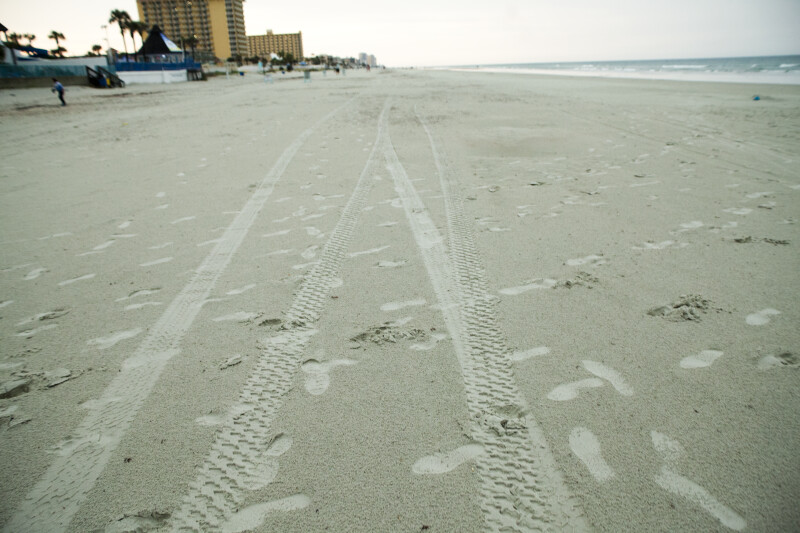A detailed photograph captures a serene beach scene, likely taken early before the area opens to visitors. The beach itself is covered in light grey to beige sand, dotted with numerous footprints and tire tracks from a vehicle that has recently traversed the area. The expansive sandy shoreline dominates the image, creating a sense of space and tranquility. 

In the upper right corner of the image, the blue ocean can be seen, its waters merging with the white sky above, hinting at the calmness of the scene. To the left, the image details several tall, light tan and yellow buildings with numerous black windows, including a prominent rectangular hotel closer to the camera and another similar structure further in the distance. Among these buildings are several palm trees, adding a tropical vibe to the setting.

Further left, there are some tent-like structures with a triangular tarp providing shade in an outdoor area, adding to the beachside amenities. The background features more buildings and trees, creating a distant, layered visual depth in the photograph. The beach itself appears deserted, lending a peaceful and almost untouched atmosphere to the scene.